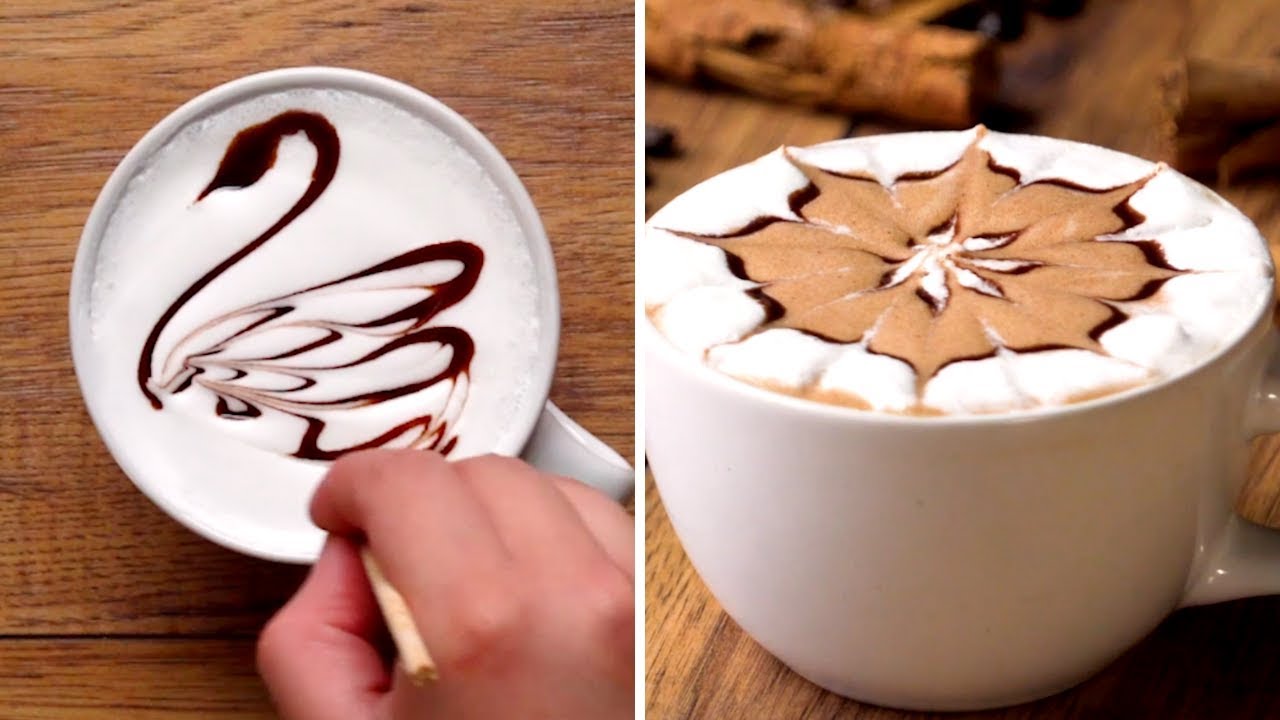The image showcases a side-by-side comparison of two intricate pieces of latte art in white mugs, set against a wooden table. On the left, a top-down view captures a delicate swan design being meticulously crafted. A hand, holding a wooden pick, is seen dragging through the creamy foam to form the swan's flowing body and elegantly curved neck. The fine lines create an impression of butterfly wings descending towards the body, with mastery and precision evident in each stroke. 

On the right, the angle shifts to a more diagonal, slightly lower perspective, focusing on a beautifully symmetrical blooming flower. This flower features eight distinct points, with the outer edges tinged a deep brown, transitioning through lighter brown inner petals, and culminating in a pure white center. Unlike the swan’s image, no hand is visible here, allowing full attention on the intricacy of the floral design. Both images rest upon a warm wooden table, emphasizing the artistry and craftsmanship involved in creating these captivating latte art masterpieces.